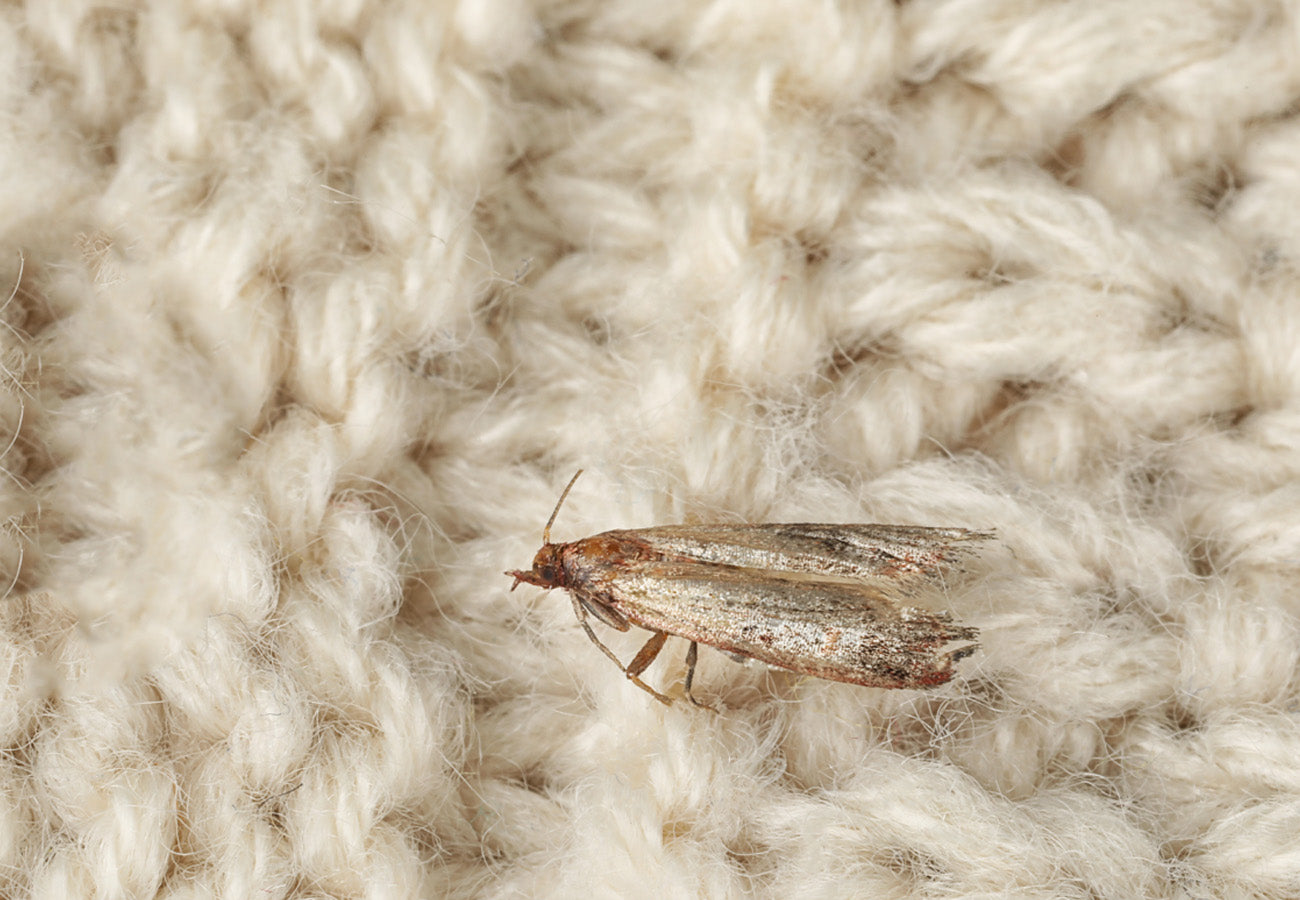This is an ultra close-up photograph capturing a small moth perched on a fuzzy knit fabric made of off-white yarn. The yarn strands show a gentle, consistent weave pattern complete with little white fibers sticking out all over, achieved through a mix of knit and purl stitches. The moth, located in the bottom right quadrant of the frame, has a body coloration that transitions from a darker reddish-brown at the head to a silvery hue towards the tips of its tattered wings. The front of its body is highlighted by black eyes and a beak-like proboscis. The moth displays two distinctly colored antennas: light gray at the top and reddish-orange at the base. Its two visible legs, also a mix of reddish-brown and light gray, cling to the knit fabric. The moth's wings, adorned with gray speckles and larger gray portions, are held tightly against its back, adding to the intricate detailing of this textured scene.